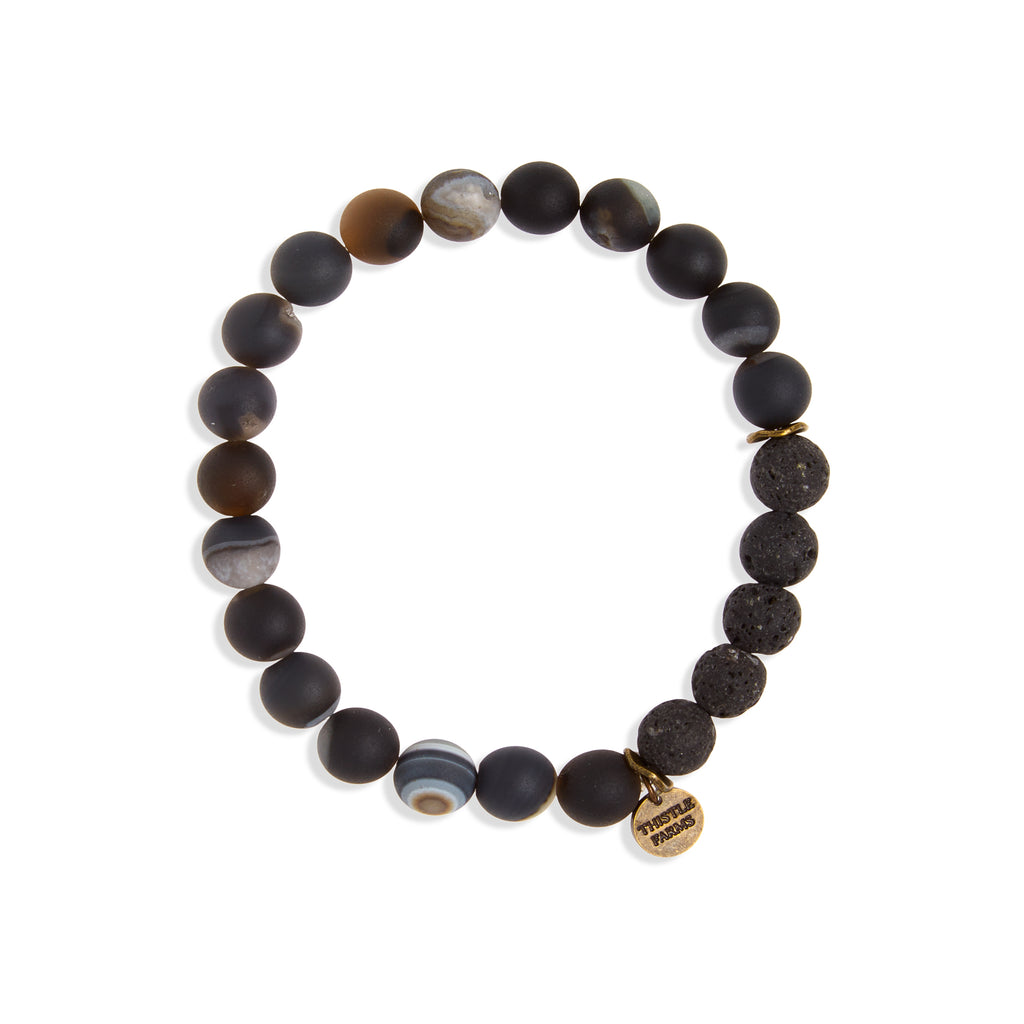This photograph captures a bracelet made primarily of dark-colored beads, featuring a mix of black, dark gray, and a few lighter or striped beads that create a muted, earthy palette. The beads, resembling stones or glass and exhibiting a variety of textures, are strung on what appears to be a stretchy cord. Two gold rings are integrated among the beads, serving as subtle spacers, with one positioned about a quarter way around from the other. Attached to one of the gold rings is an engraved gold or bronze charm, inscribed with "Thistle Farms." This charm is situated near the bottom right corner of the bracelet, adding a distinguished touch to its otherwise understated, natural look.